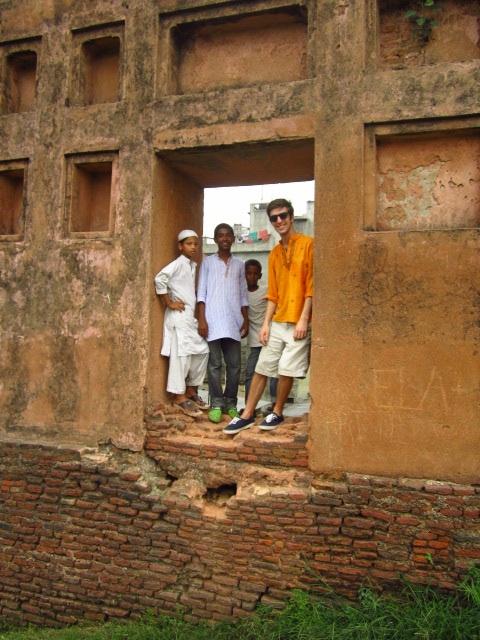In this photograph taken outside, we see a group of four people standing in a doorway of an old, terracotta-colored building. The building's wall is weathered and covered in black dirt, while its crumbling brick foundation, made up of red and brown bricks, sits beneath. Patches of green grass are peeking through at the bottom of the wall. The door itself is an empty archway with no actual door attached.

Standing in the doorway, from left to right, is a man wearing an orange shirt, white or khaki shorts, black sunglasses, and black sneakers. To his left are three boys: the first, a young child, sports a white t-shirt and jeans. Next to him is an older boy in a blue and white striped shirt that reaches mid-thigh, with jeans and green shoes. The third child, standing furthest to the left, is adorned in a white head covering, a long white tunic-style top, and loose white linen pants. The backdrop of the old building, with moss and discoloration, emphasizes the aged and worn-down condition of the structure.